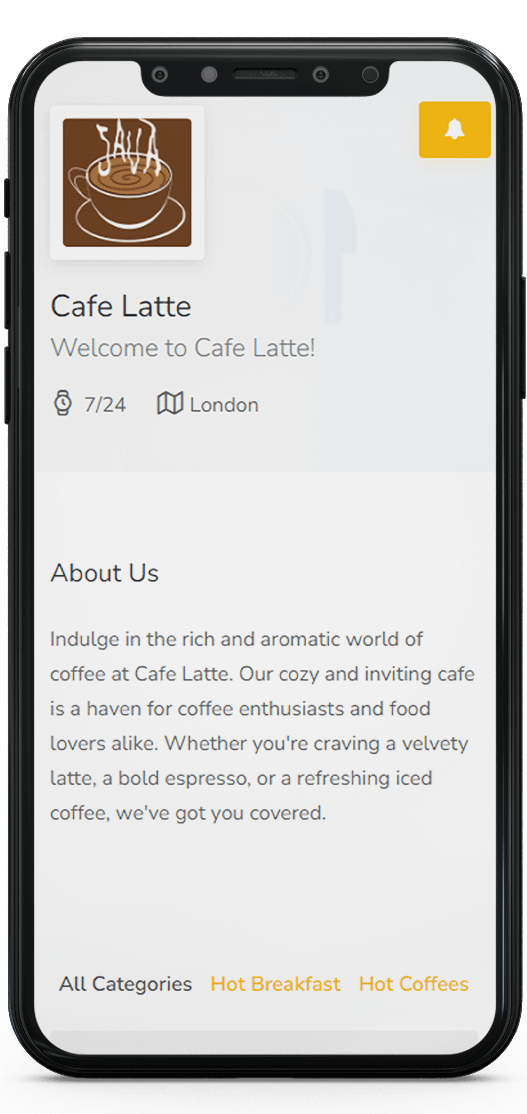Welcome to Cafe Latte! Located in the heart of London, Cafe Latte invites you to immerse yourself in the rich and aromatic world of coffee. As you open the mobile page, the Cafe Latte logo and name greet you at the top, followed by a warm welcome message dated 7-24.

Cafe Latte is designed to be a cozy and inviting haven for coffee enthusiasts and food lovers. The "About Us" section highlights the array of offerings, from velvety lattes and bold espressos to refreshing iced coffees. The cafe also specializes in serving hot breakfasts and hot coffees, catering primarily to the daytime crowd, likely those with nine-to-five jobs.

While the exact hours of operation aren't specified, it's inferred that Cafe Latte is a daytime hotspot, making it an ideal stop for morning and midday refreshments. Whether you're starting your day with a hearty breakfast or taking a break with a coffee, Cafe Latte is your go-to destination.